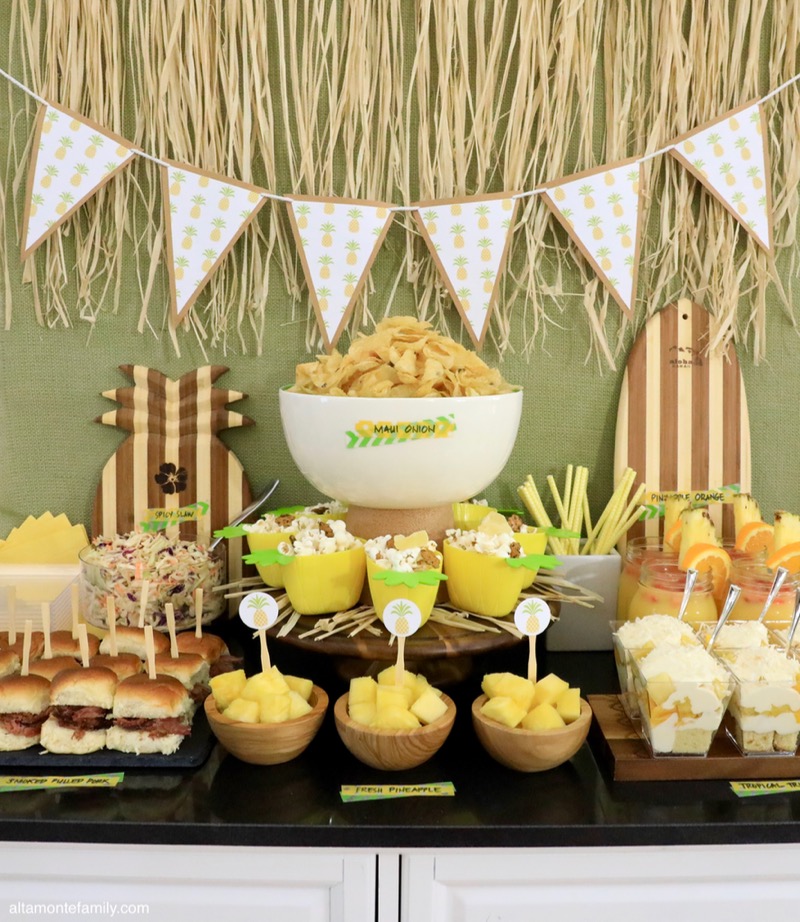A festive luau-themed party spread is beautifully arranged on a black countertop with white cabinets underneath. Hanging overhead is a cream and brown bunting paired with triangular tassel ribbons, giving off a Hawaiian vibe. Accentuating this theme, there are grass skirts draped with a decorative banner adorned with pineapples. On the right side of the arrangement, a wooden paddleboard and carved wooden pineapple add a tropical touch.

At the center of the spread is a large white bowl filled with Maui onion-flavored yellow chips. Surrounding it are various dishes, including a platter of pulled pork sliders topped with a sign labeled "sliders." In front of the sliders, three small wooden bowls are filled with pineapple chunks, each bowl featuring a card with a pineapple image. There’s also a dish labeled "spicy slaw," filled with coleslaw beneath it.

To the far right, there's a creamy, traditional tropical salad mixed with cool whip, served in clear pyramidal-shaped cups. This side also features an array of drinks, including pineapple orange beverages. The scene perfectly captures a vibrant and inviting atmosphere, ideal for a luau party.